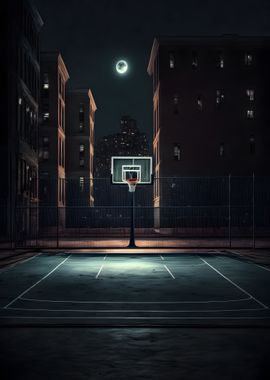The image depicts an outdoor basketball court set against a nighttime urban landscape. The court, which appears bluish-gray, occupies the foreground with its white-painted lines clearly visible. Central to the image is a standard basketball hoop, featuring an orange rim and a white net. Just behind the court, a metal fence partially obscures a series of tall, reddish-orange apartment buildings, their facades faintly illuminated by moonlight. The windows of the buildings, mostly dark, add to the overall subdued atmosphere. Above the scene, a glowing full moon dominates the sky, casting a dim, serene light over the court and giving the night an almost mystical quality. The sky transitions from an almost black hue to a dark greenish-blue gradient, enhancing the night setting.